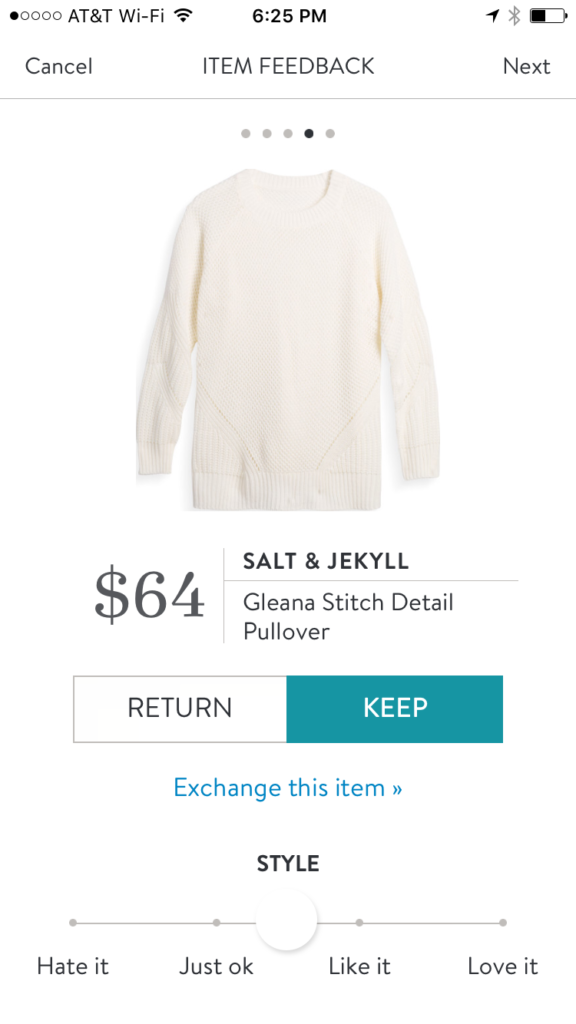This screenshot showcases an online shopping interface displayed on a smartphone, featuring a white background. Starting from the top left corner, there is a black circle followed by four white circles with black borders. Adjacent to these icons, "AT&T" is written with a Wi-Fi indicator next to it. Centrally aligned at the top of the screen, the time reads "6:25 PM." On the right side, the battery icon is displayed as half full and accompanied by the Bluetooth symbol.

Directly underneath the AT&T portion and on the left side, the word "Cancel" appears in black. In the middle section, "Item Feedback" is displayed, while on the right side, "Next" is visible, each separated by a thin gray line. Below, a navigation bar features three gray circles and one black circle. 

The main focus of the screenshot is a long-sleeved white shirt priced at $64, prominently displayed in the center. Above the shirt's name, "Salt and Jekyll," and product description, "Glenna Stitch Detail Pullover," are shown with a dividing line between them. Two action buttons are present below the description: a white "Return" button with black text on the left and a teal "Keep" button with white text on the right. 

Further down, there is a teal-highlighted option saying "Exchange this item." Below this, "Style" is written in black, followed by a line extending across the screen. This line contains four small gray dots and a larger white circle in the middle. Under each dot, options range from "Hate it" to "Love it," providing feedback choices for the item.

The composition meticulously conveys the detailed layout and interactive features of the online shopping experience.